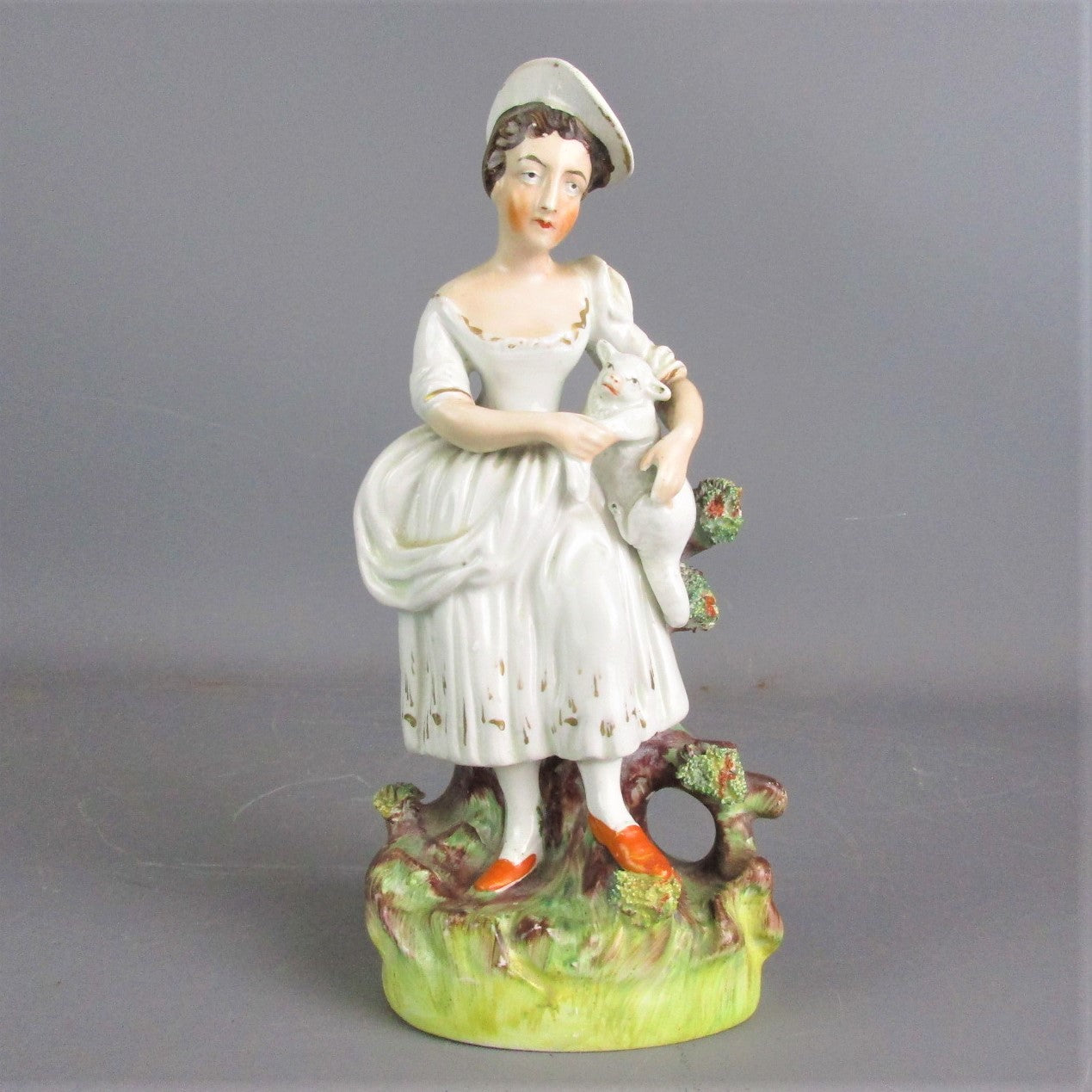This image features a porcelain figurine of a woman or mature girl standing against a gray background. She has short brown hair under a white hat that angles to the side and wears a white dress with short sleeves and a low neckline, revealing some of her shoulders and a bit of cleavage. Her dress has streaks of brown and gold accents and it flares out slightly around her thin waist, ending just above her ankles. She is adorned with very bright red lipstick and excessively rosy cheeks, giving her a striking, albeit slightly exaggerated, facial appearance. She appears to be looking to her right with an expression that suggests annoyance. Her legs are covered with white socks and she is wearing red shoes. The figurine stands on a platform designed to resemble green and brown earth, possibly depicting grass or some vegetation. In her right arm, she cradles a small lamb against her hip, with the lamb’s face visibly clear and endearing.